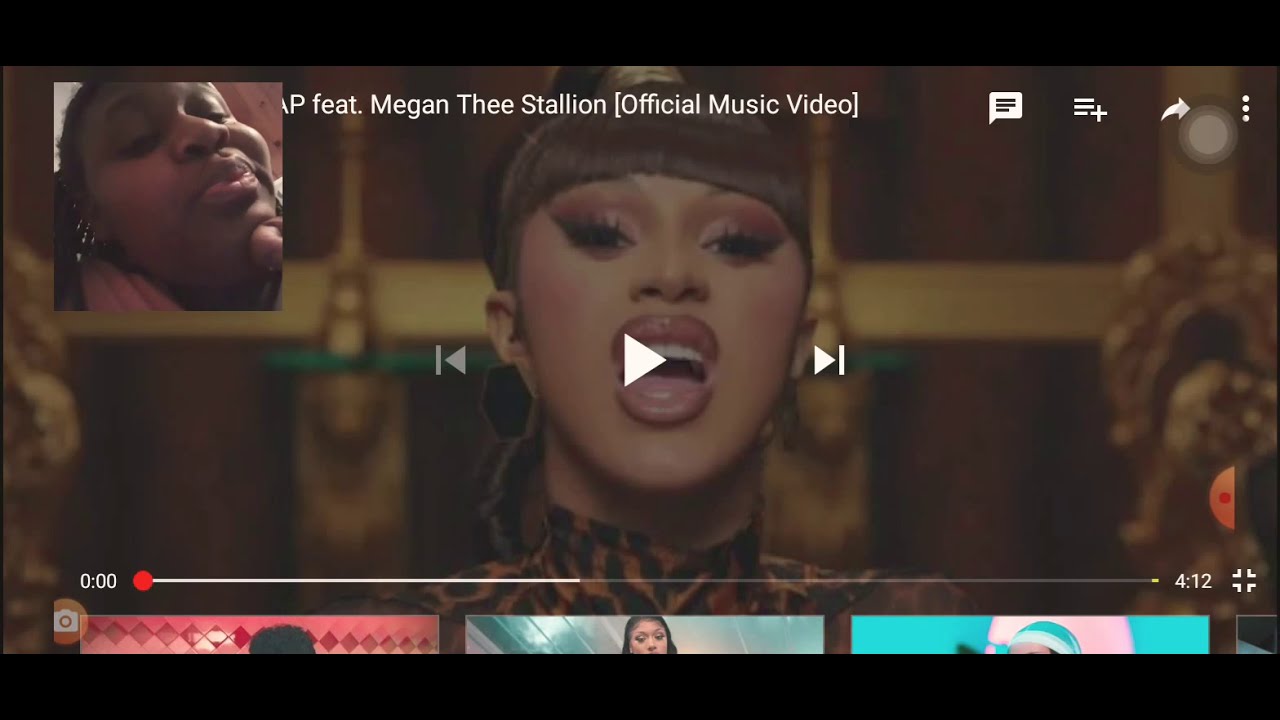This is a detailed screenshot of a phone displaying a YouTube video. The video in question appears to be "WAP" by Cardi B, featuring Megan Thee Stallion. In the still image, Cardi B's face is prominently featured, showcasing her glamorous makeup, brown hair, striking eyelashes, eyeshadow, and lipstick. She is partially visible wearing a leopard print shirt.

In the upper left-hand corner of the screen, there is a thumbnail image of an individual with African heritage, characterized by their brown skin and long curly hair styled in braids. This thumbnail partially obscures Cardi B's name.

The upper right-hand corner of the screenshot displays several standard YouTube UI elements: a captions icon (likely to enable subtitles), a hamburger menu with a plus sign (probably for adding the video to a playlist), a share button (represented by a rightward arrow), and a vertical trio of dots indicating more options.

Central to the video screen are the playback controls, including a play button flanked by back and forward buttons. Near the bottom of the screen, there is a seek bar, featuring the current playback time on the left and the total video duration on the right. A draggable red circle within the bar allows users to navigate through the video.

Finally, in the bottom right corner, a full-screen icon is present, and there are black borders at the top and bottom of the image, indicating the video might have a different aspect ratio than the phone's screen.

Overall, this detailed screenshot captures the key elements and layout of the YouTube interface as it displays the music video for "WAP."